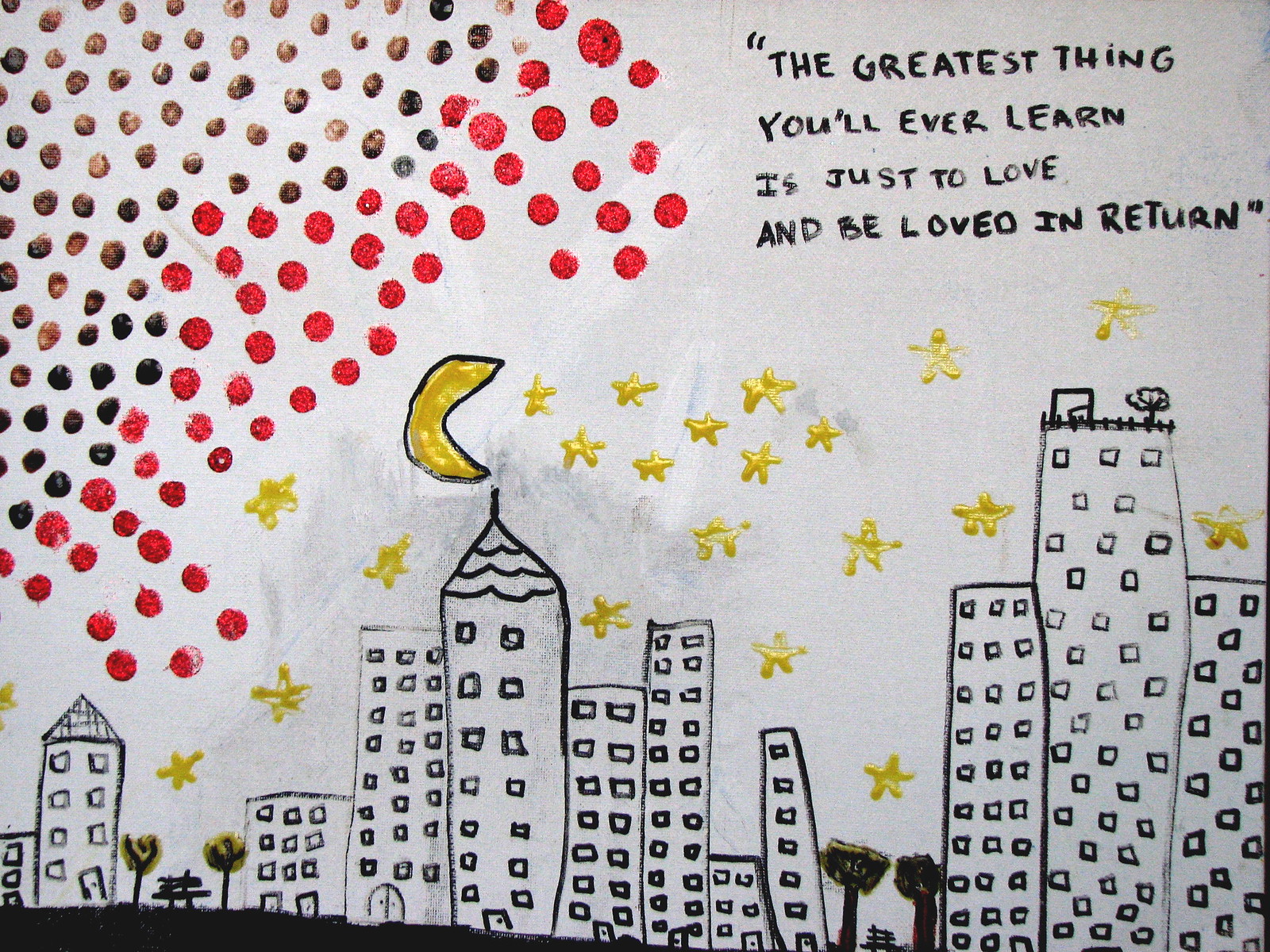The child's artwork is displayed on a rectangular piece of white paper. The image features various elements painted with different colors, creating a vibrant urban scene. In the upper left corner, an array of dots transitions from brown to red, forming an almost triangular shape. The upper right corner contains the inspirational quote, "The greatest thing you will ever learn is just to love and be loved in return," written in black paint with quotation marks. Below this, a collection of tall, rectangular buildings with square windows, some topped with slanted or pointed roofs, dominates the center. The cityscape includes at least nine buildings, with one prominent central building featuring a cone-shaped top. Interspersed between the buildings are trees with indistinguishable foliage and a small bench or table. Above the cityscape, yellow five-pointed stars and a crescent moon with black outlines illuminate the sky. The lower portion of the artwork may include additional elements like a sloping hill with more trees and another bench. Overall, the drawing captures a child's imaginative depiction of an urban landscape at night.